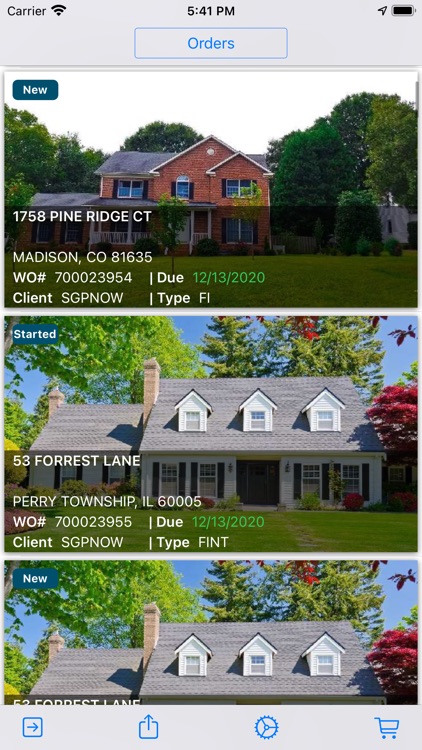The image depicts a digital interface with a light gray background, matching its light gray header at the top. In the center of the header, a bold black font displays the time, "5:41 PM." To the left of the time, the word "carrier" is written in black, accompanied by a Wi-Fi symbol, while on the right, navigation and full battery icons are visible. 

Below this header, a dark teal banner on the top left corner reads "NEW" in white text. The main section of the image features a building with black shutters on multiple windows, a gray shingled roof, and surrounded by lush, green trees and a well-manicured lawn.

At the bottom, there is a semi-transparent bar (approximately 70% opacity) with the text "1758 Pine Ridge CT" in white. Following a double space, the address "Madison, CO 81635" is displayed. Beneath the address, bold text reads "WO Number," followed by the number "700023954," in regular font.

A divider below the work order number highlights the word "Due" in bold, with the date "12/13/2020" in green. Further down, another bold label "Client" is followed by "SGP Now" in regular text. The final divider presents the bold label "Type" next to the letters "FI" or possibly "Fl" in non-bold text.